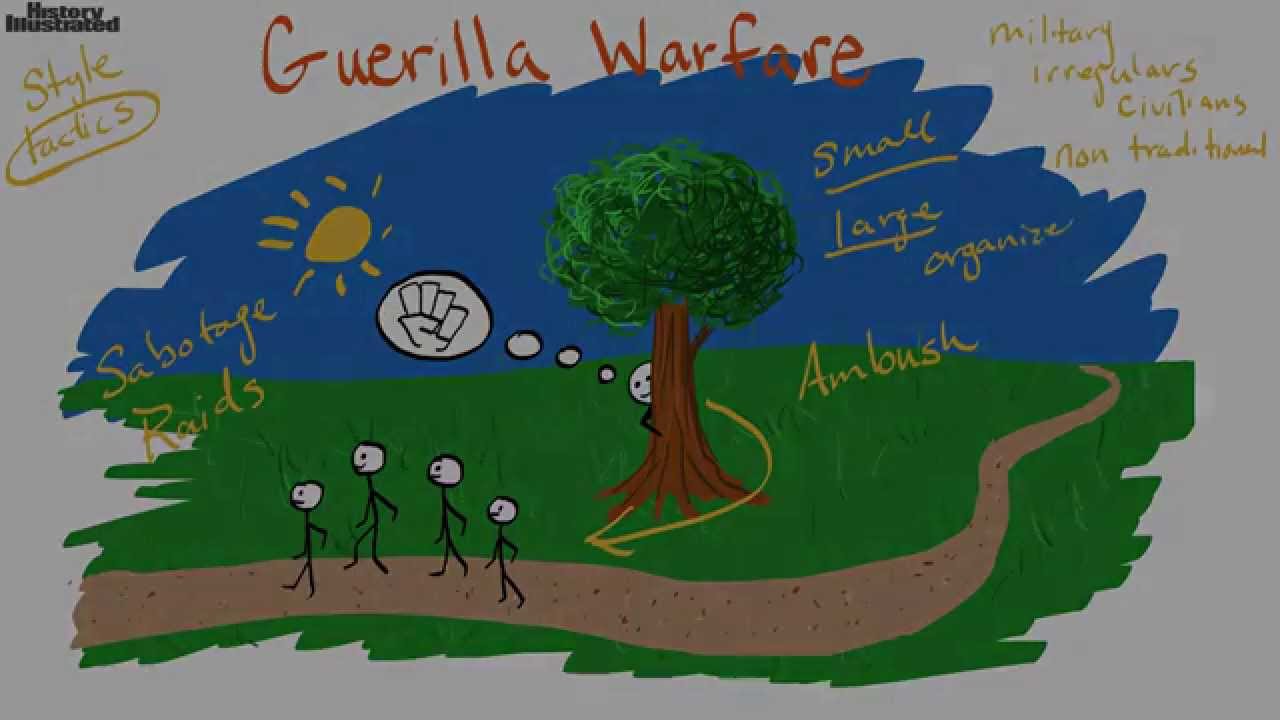This image, entitled "Guerrilla Warfare," is a cartoon-style digital drawing that resembles a simplistic, child-like whiteboard illustration. The artwork features a blue sky, green grass, a yellow sun, and a central tree with a green canopy and brown trunk. A winding brown path cuts through the scene. To the left-hand corner, the words "History Illustrated" are labeled in black text, while the title "Guerrilla Warfare" is prominently displayed in red at the top.

The image shows a stick figure hiding behind the tree, observing four other stick figures walking in a straight line along the path. The person behind the tree has a thought bubble featuring a fist, symbolizing action or conflict. Numerous terms related to guerrilla warfare tactics are scattered around the image: "style tactics" is circled to the left, and "sabotage, raids, military, irregular, civilians, non-traditional, small, large, organized, ambush" are inscribed in various locations, providing context to the scenario portrayed. The artwork uses bold, primary colors and has an amateurish, whimsical style, enhancing its instructional and illustrative quality.